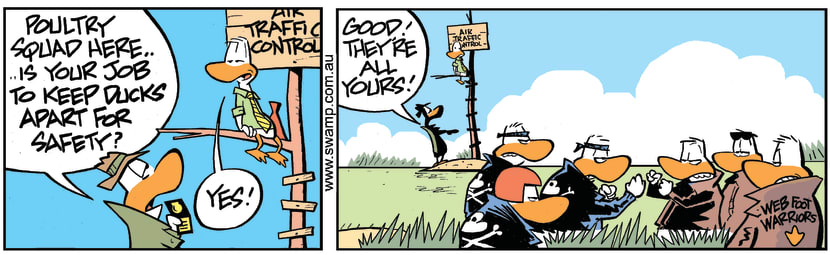This two-panel comic strip humorously depicts a chaotic "swamp PSA." In the first panel, a duck dressed as a police detective, complete with an olive green trench coat and brown fedora, presents a badge to another duck sitting atop a tree branch labeled "Air Traffic Control." The detective duck instructs, "Poultry Squad here, it's your job to keep ducks apart for safety." The second duck, looking distressed and dressed in a shirt and tie, simply responds, "Yes."

Moving to the second panel, the detective duck says, "Good, they're all yours," turning the focus to a group of six ducks in the foreground, divided into two rival gangs. On the left, a gang of ducks in black leather jackets, some with headbands and one with a helmet, sport a "skull and crossbones" emblem. Opposite them, on the right, another gang in brown detective jackets, adorned with a "Webfoot Warriors" insignia and a duck footprint, appear ready to clash. The scene captures the tension and impending conflict between the two duck factions, set against a background of grass and a blue sky with clouds, with the air traffic control duck looking bewildered by the escalation.